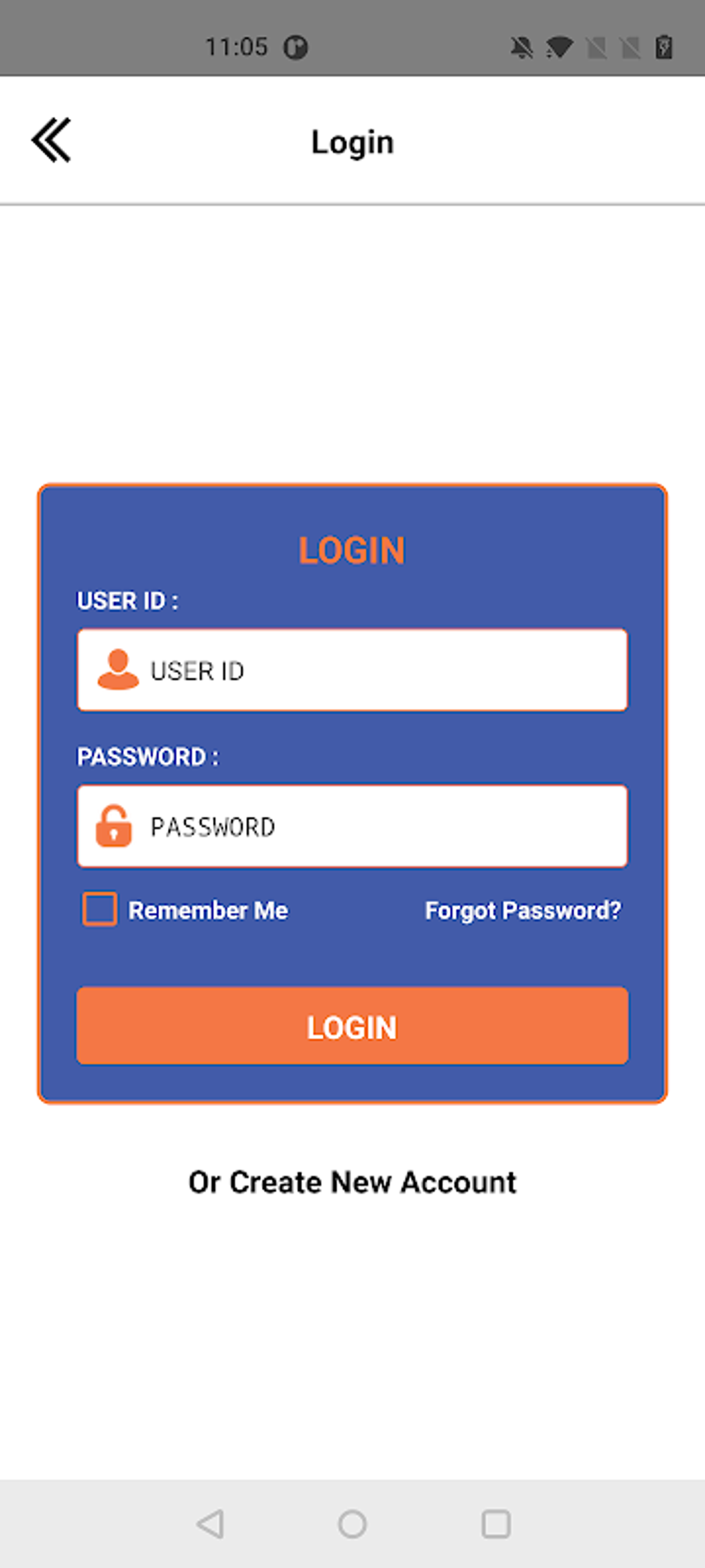This image is a screenshot of a mobile phone interface featuring a login page. The top part of the screen has a gray strip banner that displays the time as 11:05. In the upper right corner, several status icons are visible. Below the banner, there is a light gray horizontal strip with the word "Login" written in black text, centered in the image. On the far left of this strip are two left-pointing arrows.

The main section of the screenshot has a white background dominated by a pop-up login menu. This menu is square-shaped, bordered in orange, and set against a blue background. At the top of the menu, "LOGIN" is prominently displayed in orange capital letters. Below this heading, there are two input fields: one for the User ID and one for the Password. Beneath the Password field, there is an option to remember the login details, indicated by a small square outlined in orange with the label "Remember Me." To the right of this square is a link that says "Forgot Password."

Further down, there is a large orange rectangle with white text that says "LOGIN," serving as the login button. Below this button, an option to "Create New Account" is presented against the white background of the main screen. 

At the bottom of the image, a gray strip contains three navigation button icons.